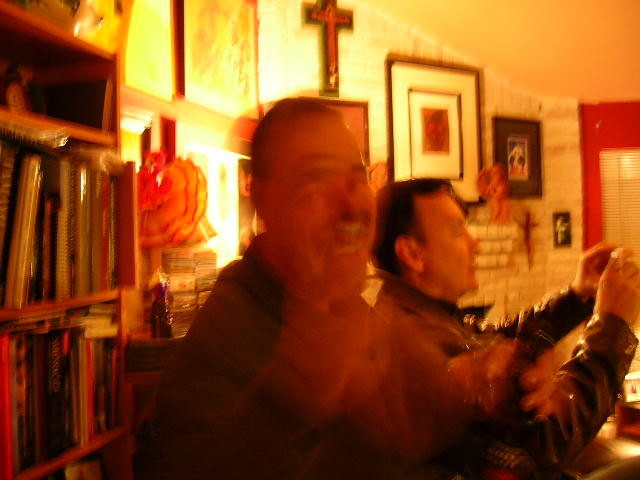In this indoor, double-exposed photograph, two men are visible amidst a brightly lit living room setting. The man on the left, appearing twice due to the double exposure, is smiling broadly at the camera, his short dark hair slightly tousled. In both exposures, his head is turned to the photographer with his eyes glancing to the left, while his left hand holds a transparent bottle of beer. He is wearing a dark-colored jacket, possibly red or black. The other man, located on the right, is staring to the right side of the image. He has short black hair, and is dressed in a black leather jacket. His hands are held in a triangular shape, palms together, potentially holding a camera. 

The background is enriched with several details: a tall bookshelf filled with books and notebooks, a white brick shelf adorned with statues, and a framed artwork with thin brown borders and a red center. There is also a cross mounted on the wall above the piece of art. Another detail includes a red wall fitted with a window, partially covered by white blinds. The brightly lit setting, double exposure, and arrangement of elements create an intricate, layered scene.